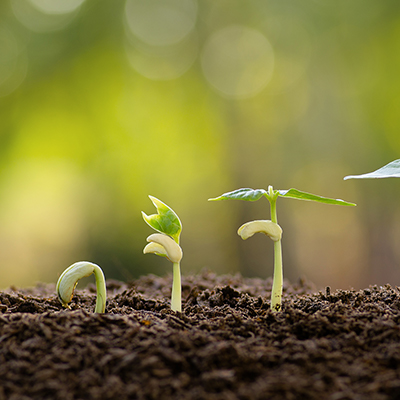The photograph captures a close-up view of three plant seedlings at different stages of growth, emerging from dark, freshly-tilled, nutrient-rich soil. On the left, the first stage shows a small seedling, bent over with its leaves unopened, barely poking through the dirt. The middle seedling represents the second stage of growth, standing tall with two leaves midway through opening, resembling tiny green horns or limbs. The third and final stage is depicted on the right, where the stem is straight and taller, approximately five to six inches, with fully developed, wide-open leaves. The background features a blurred, watermelon-green hue, ensuring all attention remains on the progressing seedlings. Additionally, there are subtle white dots that appear to be light refracting in the background, contributing to the crisp and clear focus on the plants in the foreground.